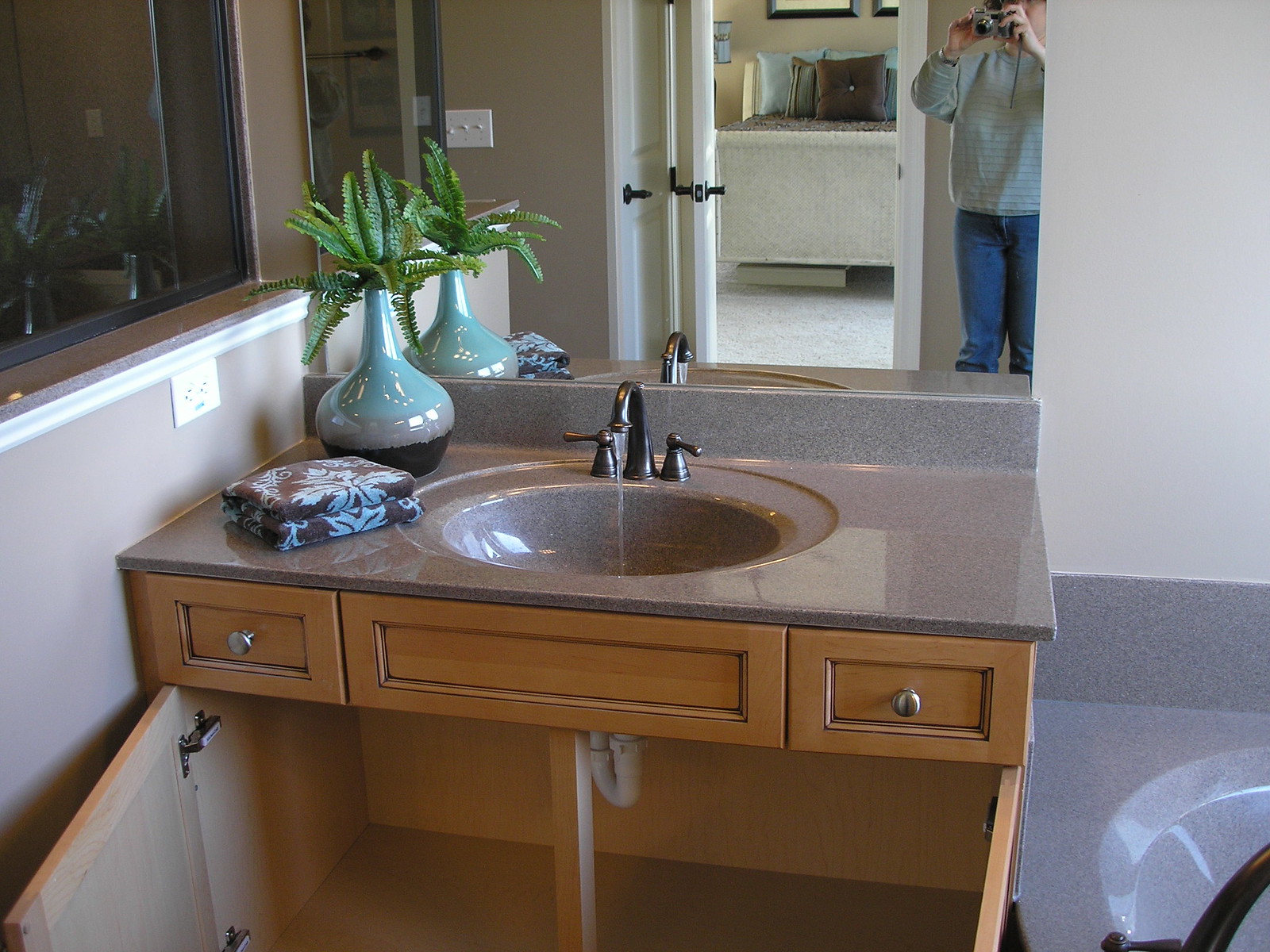Here is a clear and detailed photograph of a modern bathroom. The sink features a striking basin and countertop made of brownish-pink and gray marble tile. The central faucet is a deep bronze or copper shade, adding an elegant touch. On the sink's countertop, there's a multi-toned ceramic plant holder that transitions from black at the base to gray in the middle, and finally to sky blue at the top, housing a vibrant green plant.

Next to the sink, a set of black blankets decorated with blue petaled flowers are neatly placed. The area beneath the sink is minimalistic, with only plumbing connectors visible, maintaining a clean look.

The bathroom floor is gray, contrasting softly with the off-white walls. Through an open doorway, another room is visible, featuring a cream-colored bed adorned with brown and blue pillows. A person dressed in blue jeans and a green and white shirt is captured in the act of taking a photograph, adding a candid, lively element to the scene.